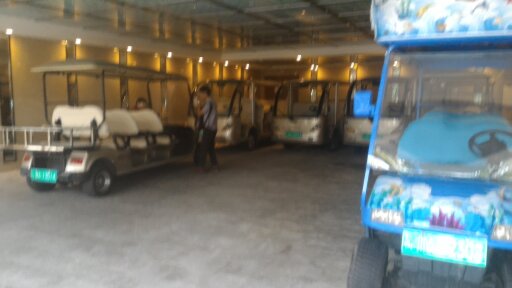This slightly blurry, color photograph, oriented in landscape, captures a collection of golf buggies inside a spacious, resort-like garage with an exposed beam roof and recessed lighting. At least six or seven buggies are visible, each detailed meticulously. The buggies in the background, mostly gold in color, are arranged in neat rows, equipped with beige seats, an open top with a beige roof, and large racks at the back for holding golf clubs or luggage. One of these buggies, positioned on the left, is facing away from the viewer, with a discernible individual seated in the driver's seat and another person standing beside it.

Dominating the right side of the image is a distinctive buggy, partially cut off, featuring a striking blue pattern with white accents and an ocean reef design. Its black left wheel is angled towards us, and through its windshield, the black steering wheel and blue seats can be seen. Intriguingly, this blue buggy also has a plate on the front, although the inscription isn't readable due to the photo's blurriness. The garage floor is illuminated by numerous spotlights positioned along the left and right sides, casting yellow cones of light downwards, adding a warm glow to the scene.